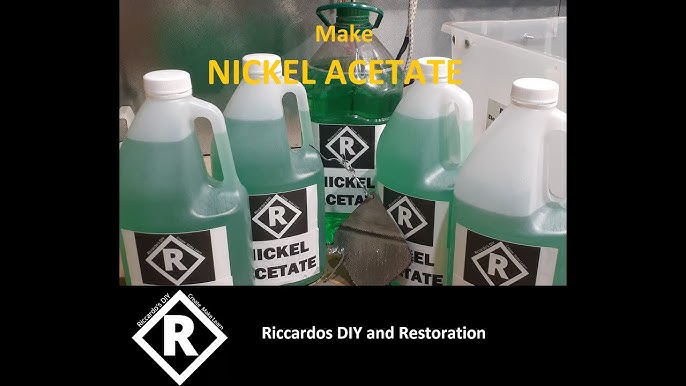This image, featuring an instructional graphic, showcases Ricardo's DIY and Restoration's process for creating nickel acetate. The illustration is encased in a U-shaped black border, highlighting the central content. At the bottom, a diamond-shaped logo with a prominent 'R' is visible, alongside the text "Ricardo's DIY and Restoration." The main image displays five bottles, four of which are plastic containers filled with green liquid, labeled "nickel acetate" and adorned with Ricardo's logo. In the background, there is a larger, approximately two-gallon glass jug containing the same green liquid, marked similarly. Overlaying the image in yellow letters is the title, "Make Nickel Acetate," indicating that the purpose of this visual is to guide users through the process of creating nickel acetate. The detailed setup suggests the image might accompany an article or tutorial on the subject.